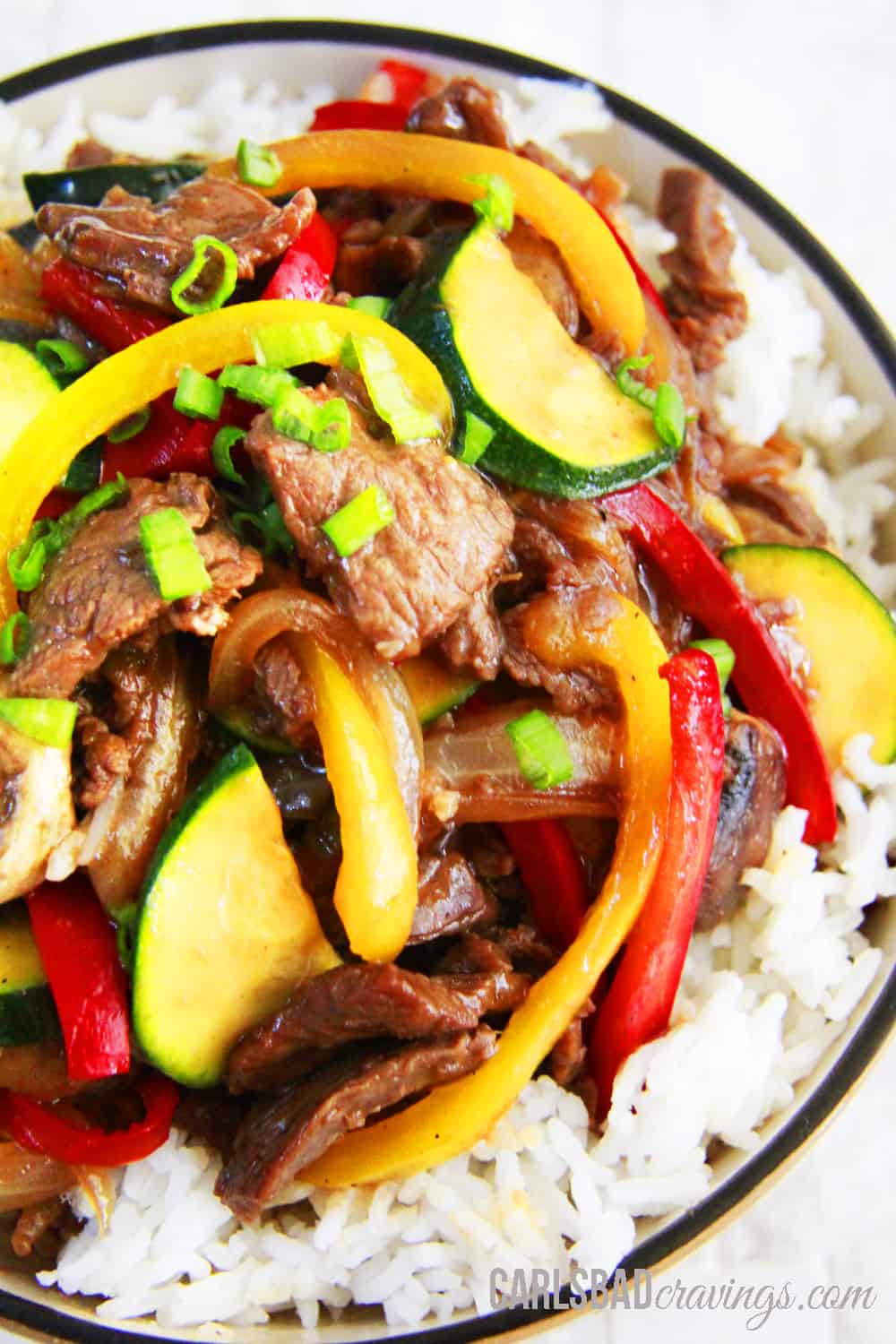The image features a visually appealing, close-up portrait of a vibrant and appetizing meal set against a clean white background. The centerpiece is a white bowl with a distinct black and yellow border around the top edge. The bowl is generously filled with a bed of fluffy white rice, topped with an assortment of colorful, fresh ingredients. 

Prominently displayed on top is a serving of savory meat, likely either beef or chicken, which appears to be coated in a delicious teriyaki sauce. Accompanying the meat are an array of sliced vegetables, including red and yellow bell peppers, zucchini, and mushrooms, adding both color and nutritional balance to the dish. Garnishing the meal are finely sliced green onions and possibly cilantro or parsley, enhancing its visual appeal and flavor profile.

The presentation suggests a healthy and well-prepared Asian-inspired dish, possibly created for promotional purposes as indicated by the text "carlsbadcravings.com" subtly placed in light gray in the lower right-hand corner of the image.